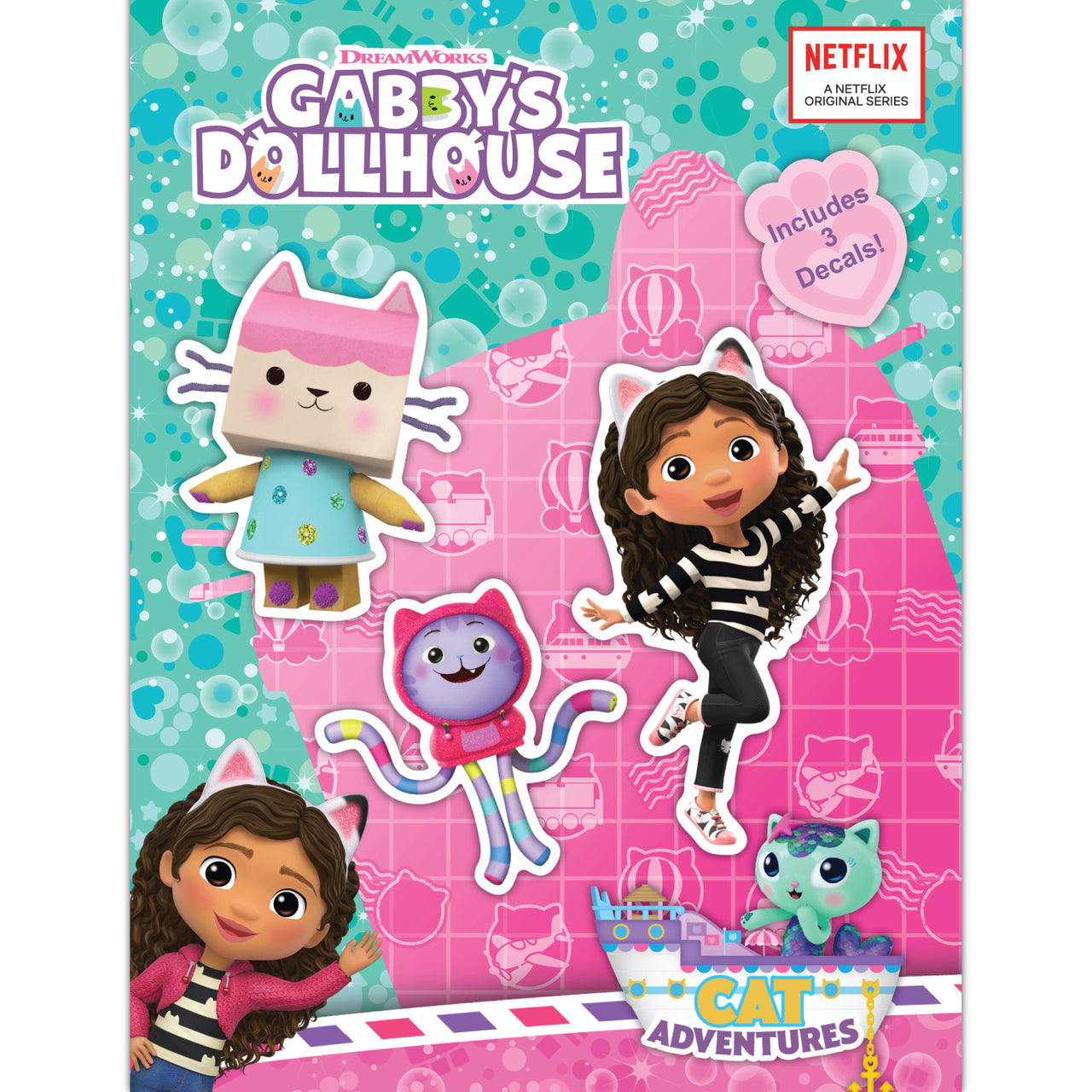This is a promotional poster for DreamWorks' series "Gabby's Dollhouse," prominently featuring vibrant colors like purple, orange, aqua blue, regular blue, and pink. At the top left corner, "DreamWorks" is written in pink letters, and below it, "Gabby's Dollhouse" is prominently displayed in bold white letters with purple outlines, with playful cats peeking out in colors blue, green, orange, and pink. In the top right corner, there is a red rectangle with white filling containing the text "Netflix" in red, and underneath it in black, it reads "a Netflix Original Series." Further down, a pink heart emblem indicates, "Includes three decals." The bottom of the poster features the phrase "Cat Adventures," with "Cat" in yellow and "Adventures" in purple. The focal point is a girl with long brown hair, dressed in black and white striped shirts. She is wearing cat ears and variations include a pink cardigan, light denim pants for one, and dark pants for the other. Among the characters, there are three distinctive cats—a cat with a bag resembling a cat face, dressed in a blue polka dot dress, a cat in a hoodie, and a cat adventuring in a ship.